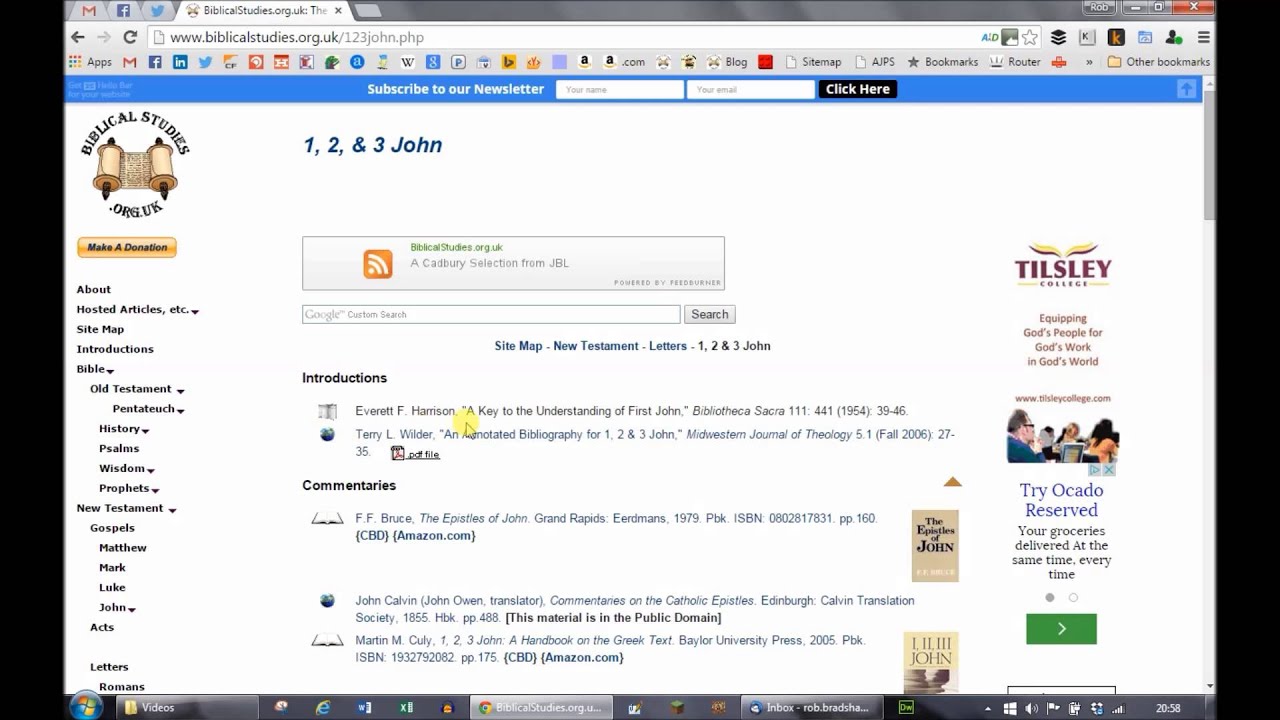A user is browsing a web page on biblicalstudies.org.uk, specifically at the address www.biblicalstudies.org.uk/123john.php. The browser displays several other open tabs, including Gmail, Facebook, and TwitterX. 

At the top of the biblical studies page is a bright blue banner featuring a call-to-action message in the center: "Subscribe to our newsletter." Below this prompt are white input boxes for "First Name" and "Email," accompanied by a black "Click here" button.

In the left corner beneath the banner, set against a white background, is the site's logo—a scroll image beside the text "biblicalstudies.org.uk" in bold black letters. Adjacent to this, in bright blue text, reads "1, 2, and 3 John."

Scrolling down the left-hand side, under the logo and site name, a yellow box with black text encourages visitors to "Make a donation." Below this box is a vertical navigation menu listing categories such as "Hosted Articles," "Sitemap," and "Introductions." More specific subcategories follow, including distinct sections for the "Old Testament" and the "New Testament," with further indented subcategories under each, like "Pentateuch," "History," and "Wisdom" for the Old Testament, and "Gospels," "Acts," and "Letters" for the New Testament.

The primary content of the page focuses on the New Testament letters 1, 2, and 3 John, with various introductions and commentaries available for readers.